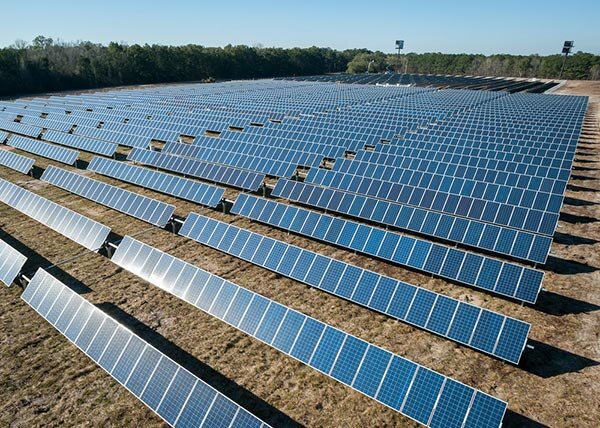This photograph captures a large, rectangular solar farm with countless rows of dark blue, rectangular solar panels. These panels, meticulously aligned in parallel formations, are slightly tilted upwards to maximize sunlight absorption. The ground beneath the panels is covered in dark brown soil. The panels catch the sunlight, casting visible shadows to their right. Encircling the solar farm, a tree line with dark green foliage frames the background, while a clear, light blue sky stretches above, adding to the serene and structured scene. The panels themselves exhibit slim, geometric frames with thin grey lines crisscrossing their surfaces, emphasizing the extensive and methodically arranged layout of this vast renewable energy site.